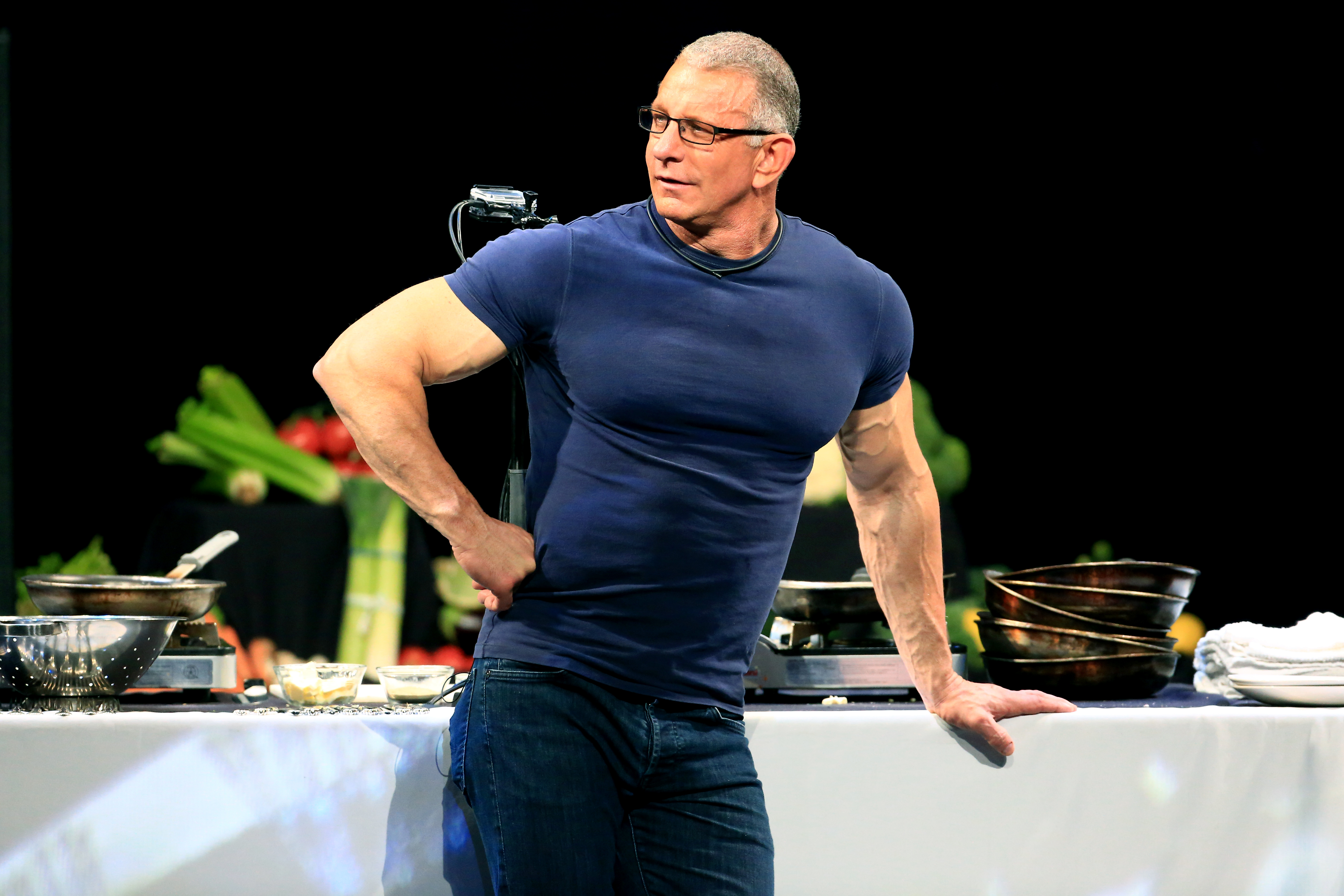The photograph, a rectangular indoor shot measuring approximately six inches wide by four inches tall, features a strikingly muscular elderly Caucasian man standing mid-thigh and up. Set against a predominantly black background that covers three-quarters of the image from the top, the lower quarter showcases a table dressed in a white tablecloth. Arrayed on the table are various kitchen items like mixing bowls, a frying pan, a hot plate, a colander, and an assortment of green fruits and red vegetables.

The man, identified as a familiar chef renowned within cooking circles who may be married to the professional wrestler Gail Kim, poses confidently with his left arm resting on the table for support. His right arm is bent at the elbow, his fist positioned authoritatively on his waist. Clad in a skin-tight, short-sleeved dark navy blue shirt that molds to his well-defined biceps and pectoral muscles, he also wears blue jeans. His mostly white hair, speckled with gray and cut short, complements his thin-rimmed black glasses. Gazing to the left, his slightly open mouth suggests he might be in mid-conversation or about to speak.